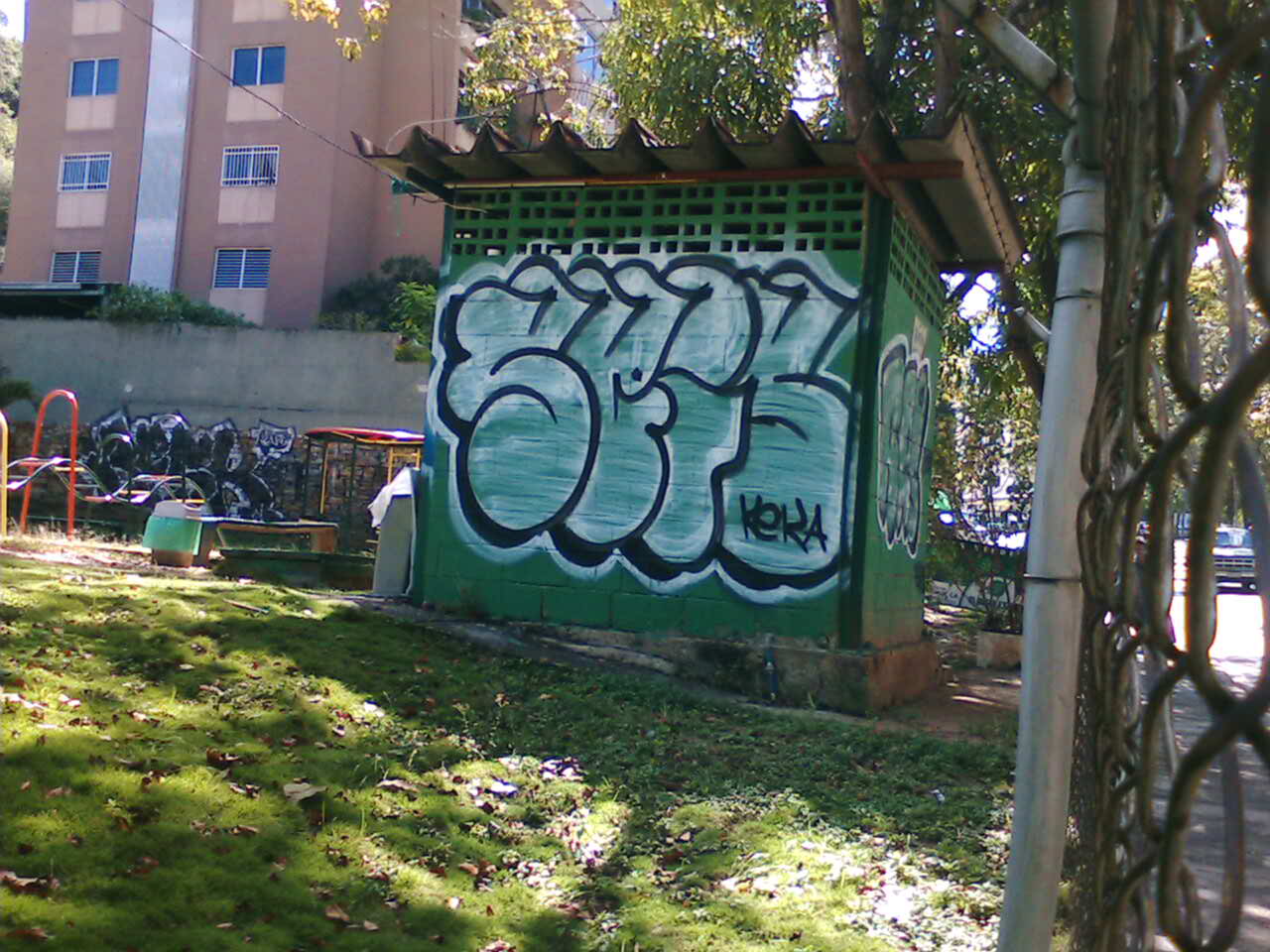The image depicts an outdoor urban setting, centered around a graffitied green hut or storage shed located in a playground. The shed, potentially serving as the back of a bathroom, features large puffy graffiti letters. Although the complete letters are not legible, the lower right-hand side contains the characters "K-E-K-A" in light green with a black outline. The playground is strewn with brown dead leaves on green grass, bordered by a chain-link fence to the left. Adjacent to the left of the green shed is a short gray concrete wall, which itself is heavily graffitied. Beyond this wall, we see a tall, brown, cement-colored building that appears to be an apartment complex with at least four to five floors, each adorned with a set of windows. Metal rectangular structures run vertically between the windows from the top to the bottom. Overhanging the gray wall are some trees and bushes, adding greenery to the scene. In summary, the graffiti-laden hut, playground foliage, and towering background building create a vivid snapshot of urban life.